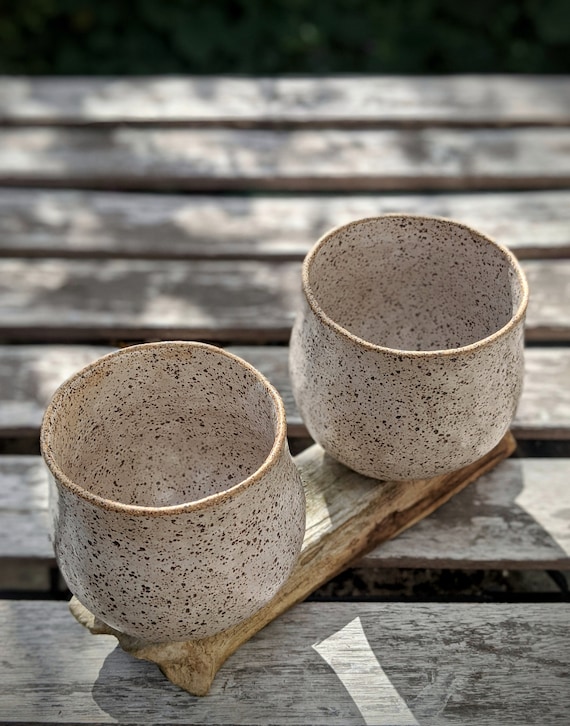The photograph captures a close-up of two small, handleless cups, each white speckled with brownish-beige, resting on a piece of driftwood-styled wood used as a tray. This setup is placed on a rustic, weathered wooden surface with noticeable spaces between the planks, suggestive of a picnic table or similar wood structure. The cups appear handcrafted with subtle irregularities, enhancing their natural, artisanal feel. The backdrop features blurred foliage, casting leaf shadows onto the table, evoking a relaxed, sunlit outdoor ambiance.